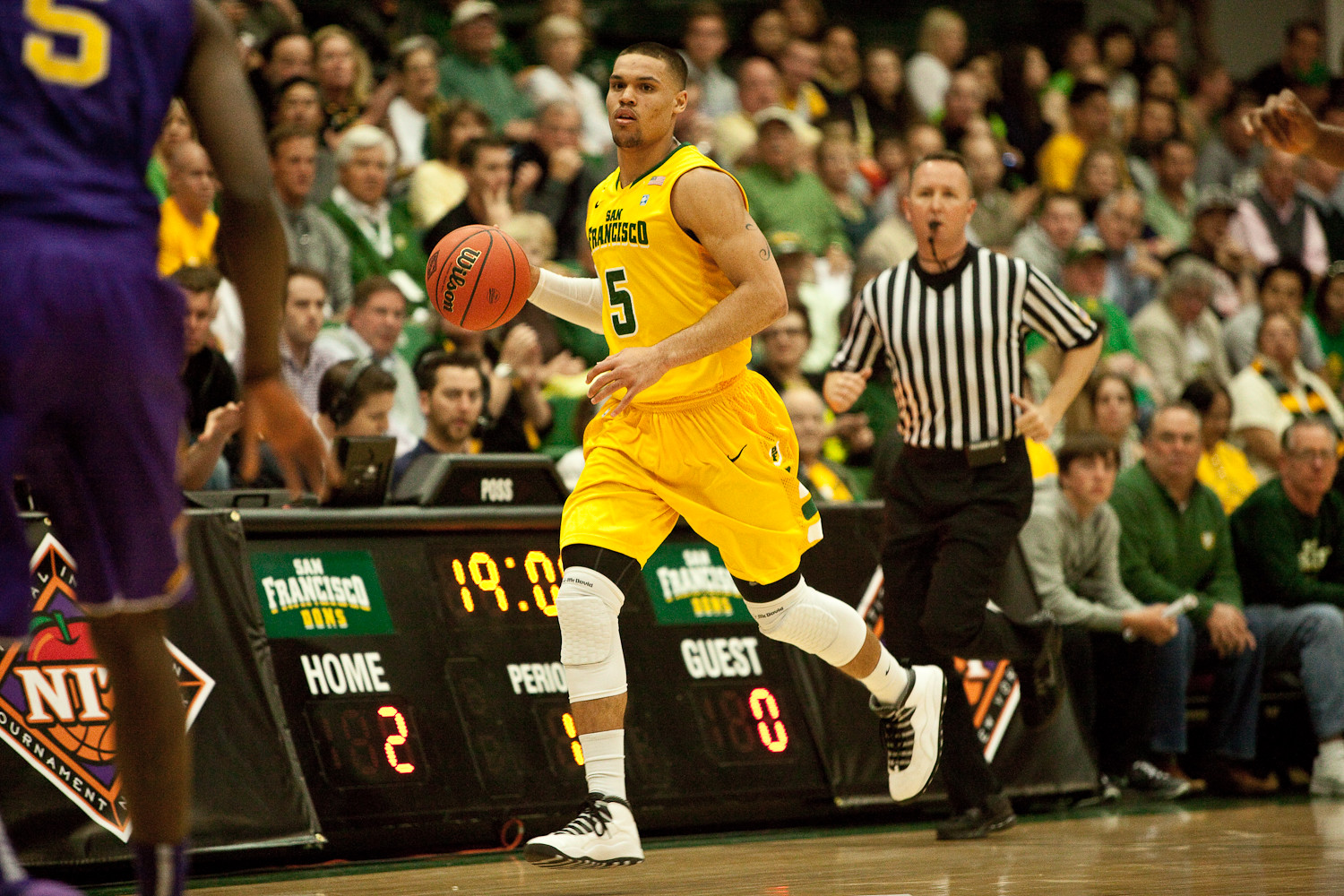In this vibrant photograph of a professional basketball game, a player in a yellow San Francisco Suns uniform with the number 5 prominently displayed is captured mid-action, dribbling the ball. The basketball, displaying the Wilson logo, is a classic orange and black. Close behind him, a referee in a white and black vertically striped shirt with a whistle in his mouth keeps pace, while to the left, partially cropped from the frame, stands an opposing player in a purple uniform, poised to intercept. The digital scoreboard on the floor indicates the Suns leading with a score of Home 2, Guest 0, with 19 minutes remaining on the clock. In the blurred backdrop, an enthusiastic crowd watches the unfolding drama.